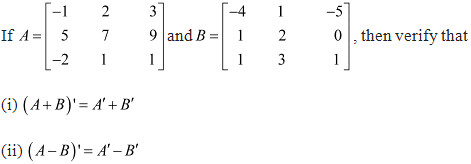The image depicts a mathematical problem involving matrix operations. The problem features two matrices named 'A' and 'B', each organized in a 3x3 grid format, containing integers in specific rows and columns. The caption for the image reads:

"Given matrices A and B, both structured as 3x3 grids with integer elements, verify the following properties:

1. \( A + B = A + B \)
2. \( (A - B) = A - B \)

The task requires solving the problem by applying the formulas to the integers arranged in the respective rows and columns of matrices A and B."

This caption serves to elaborate on the visual content, highlighting the verification of matrix addition and subtraction identities.